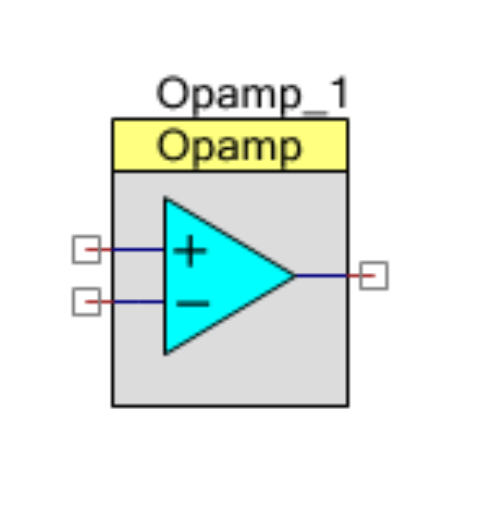The image is a slightly blurry depiction of a circuit diagram set against a solid white background. Central to the image is a vertically oriented, light gray rectangle. At the top of this gray rectangle, there is a horizontal yellow rectangle containing the fuzzy black text "OPAMP." Directly above this yellow section, the clearer black text "OPAMP_1" is written. Below the yellow rectangle, within the gray rectangle, sits a light blue triangle pointed to the right. This triangle features a plus sign at its top vertex and a minus sign at its bottom vertex. Extending from these signs, blue lines emerge from both the plus and minus signs. These lines turn red as they exit the gray rectangle and intersect with small gray squares. The diagram details show connections indicative of an operational amplifier circuit, represented by the "OPAMP" labels and the symbolic triangle.